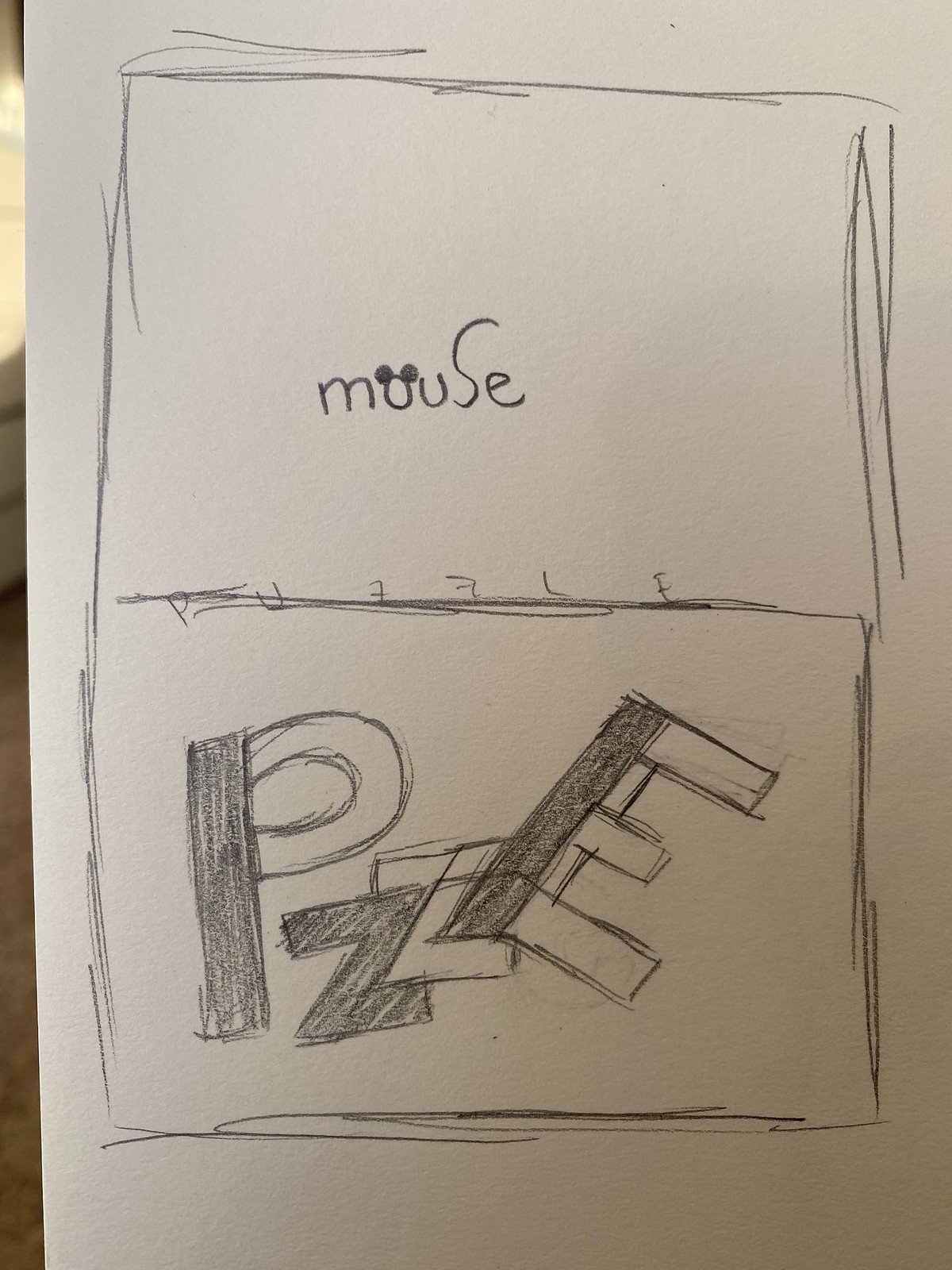A piece of plain white paper features a meticulous pencil drawing. Central to the composition is a tall, slender rectangle bisected by a horizontal line. Along this line, the word "puzzles" is written in neat, uniform letters. Positioned at the top of the rectangle is the word "mouse." The letter 'O' in "mouse" is uniquely stylized, with two small round circles adorning each side of the 'O'. The 'S' extends dramatically upwards, towering at more than twice the height of the surrounding letters. At the bottom section of the rectangle, the letters "P, Z, Z, E" are inscribed. The straight line of the 'P' is fully shaded while its loop remains uncolored. The first 'Z' is filled in with pencil, contrasting with the second 'Z' which remains unshaded. Lastly, the vertical line at the back of the 'E' is shaded, while the horizontal strokes and remaining section are not.